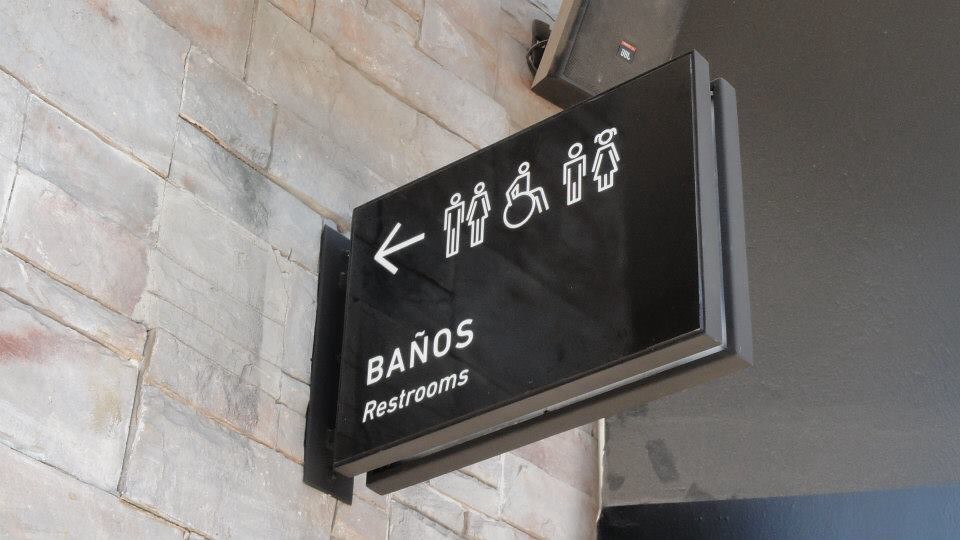The photograph depicts a public bathroom sign on a light-colored brick wall. The image is taken from the perspective of someone standing on the ground looking slightly upwards. The left side features a tall, light-colored brick and stone wall, while the right side shows a white wall with a hint of blue at the bottom and a gray speaker at the top. Centrally positioned on the wall is a black sign extending from a bracket on its left. The sign displays clear white text stating "Baños Restroom" with a left-pointing arrow. It also includes pictograms of a man and woman, a person in a wheelchair, and smaller figures of a boy and girl, indicating the restroom's accessibility and family-friendly nature. This detailed sign provides direction to restrooms located inside the building.